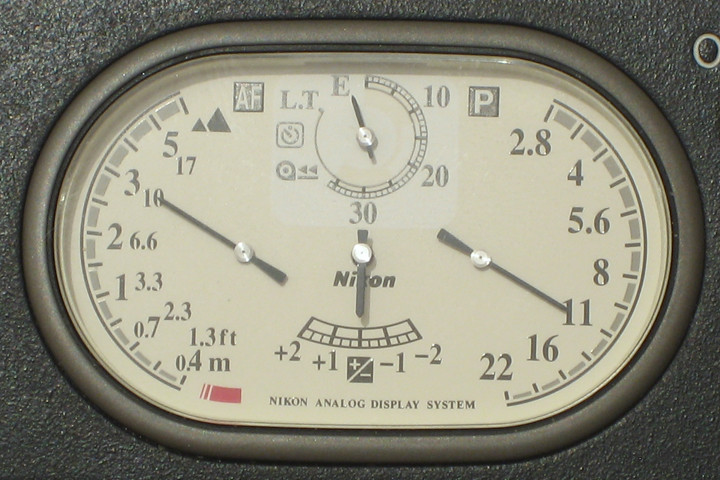This detailed description is intended to paint a comprehensive picture of the Nikon analog display system meter for those who cannot see the image.

---

Image Caption: 

The photo showcases a Nikon analog display system featuring an intricate array of dials and indicators. The main display area is an oval-shaped dial with rounded sides and flat top and bottom edges. Prominently, there are two large semi-circular dials positioned on the left and right sides.

The left dial includes a small black hand pointing to various measurements. At the bottom, it is labeled "1.3 FT" (feet) and below that, "0.4 M" (meters). This suggests the dial might be measuring some form of distance or pressure. The increments on this dial are somewhat unconventional, marked at 0.4, 0.7, 1, 2, and 3 meters from bottom to top. At the upper left, there is an icon depicting two mountain-like peaks, possibly indicating a terrain measurement or altitude-related function. Further, a section towards the bottom of this dial is highlighted in red, perhaps serving as a warning area for critical ranges.

The right semi-circular dial features a prominent white "P" inside a black square at its upper right corner. This dial is marked with values that appear to follow a geometric sequence: 2.8, 4, 5.6, 8, 11, 16, and 22. These values are printed in black and might correspond to settings or a specific type of measurement.

Centrally located between the large dials are two smaller dials. The upper center dial is perfectly round, featuring a small black hand, and is marked with values "E," "10," "20," "30," along with some circular icons and "L.T." Below this is another smaller semi-circular dial, with the Nikon logo situated just beneath it. This dial has a black hand pointing to markings from plus 2 through minus 2, perhaps for fine-tuning or balance adjustments.

Overall, this Nikon analog display system appears to be a highly specialized instrument, incorporating various measurement dials and indicators, likely used in a precise technical or scientific context.